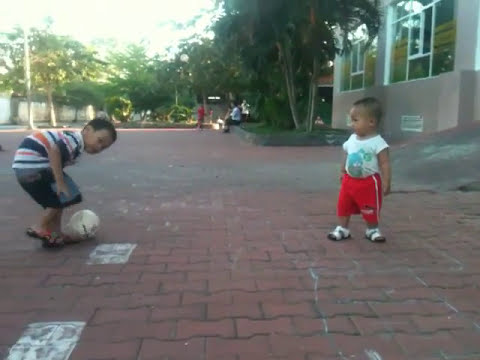In this vibrant outdoor scene, two young Asian children are delightfully engaged in play on a surface of red brick pavers. The smaller of the two, likely a toddler still in diapers, is dressed in white sandals, red shorts, and a white T-shirt featuring a cartoon character. This child is on the right side of the image, standing with a slight poofy belly peeking over the shorts. To the left, an older boy, estimated to be between five and seven years old, is captured bending towards a white ball on the ground while glancing back at the camera. He wears a striped polo shirt with colors of white, black, and orange, paired with blue jean shorts and sandals. The bottom two-thirds of the image focuses on the children at ground level, showcasing the well-worn red brick pavers, some with faded white lines. In the background, bathed in sunlight, is a bustling scene with trees and an adult figure near what seems to be a building or apartment with pinkish-gray stone walls and various windows. People can be seen sitting along a bench, adding a sense of community and liveliness to the picturesque setting.